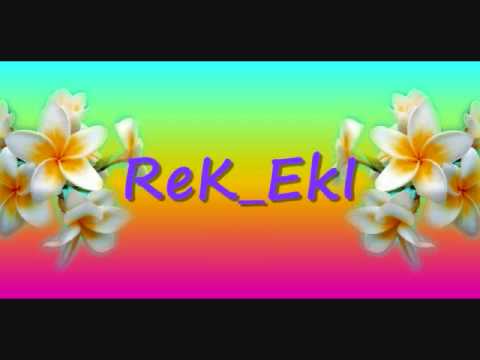The image features a widescreen, letterboxed design with a vibrant gradient background transitioning from light turquoise at the top, through green, yellow, and orange, and ending in bright pink at the bottom. Flanking both the left and right sides are clusters of white, tropical-looking flowers, each with five oval-shaped petals forming star-like shapes and centered around yellow or orange circles. At the center of the image, in prominent purple text, reads "R-E-K underscore E-K-L," with a pattern of alternating uppercase and lowercase letters. The overall design appears to be a logo or a computer graphic composition.